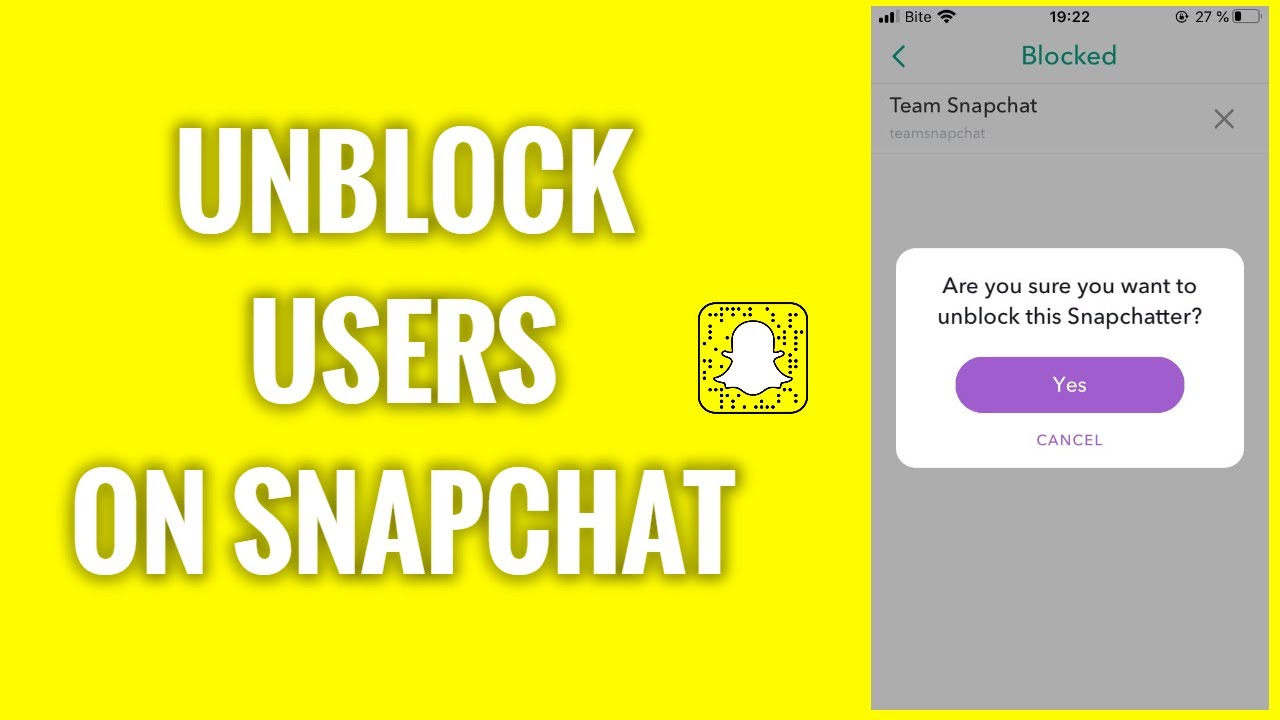The image serves as an instructional guide on how to unblock users on Snapchat. On the left side, a bold and capitalized title in white font reads "UNBLOCK USERS ON SNAPCHAT," set against a vivid yellow background. Adjacent to the title on the right is the iconic Snapchat logo—a simplistic, white ghost figure surrounded by a border that resembles Braille markings.

Further to the right, a screenshot from a smartphone is visible. The screenshot features a pop-up window with the message, "Are you sure you want to unblock this Snapchatter?" offering two options: "Yes" and "Cancel." This visual demonstrates the steps a user might take to remove someone from their block list on the Snapchat app.

Overall, the image effectively functions as a visual tutorial for unblocking users on Snapchat, showcasing both the title on the left and a practical example of the unblocking process on the right.